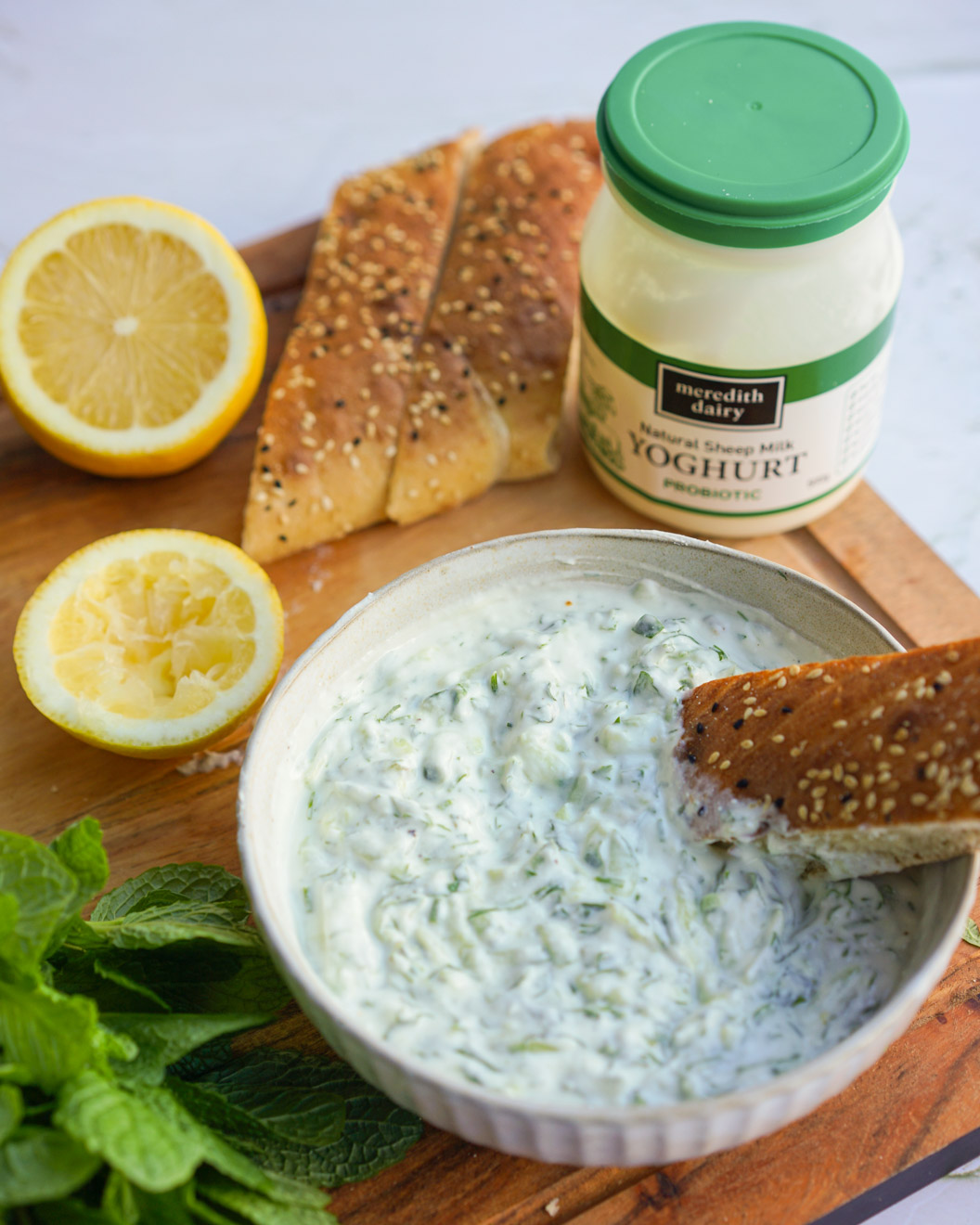This photo showcases a well-prepared yogurt dip arranged on a wooden cutting board. The main highlight is a porcelain bowl filled with a creamy, white yogurt dip, possibly a dill-infused tzatziki sauce. A piece of poppy seed and sesame seed bread is dipped into the yogurt mixture, emphasizing the dip's use in the meal. To the left, a bright yellow lemon is neatly sliced in half, hinting at its use in the dip’s preparation. Two additional slices of toasted sesame and poppy seed bread are nearby. A green-lidded canister of Meredith Dairy Natural Sheep Milk Yogurt Probiotic, used to make the dip, is prominently featured. Bright green leafy herbs, potentially dill or mint, are placed in the bottom left corner, adding a fresh essence to the setup. The wooden cutting board provides a rustic base, while a clean white background enhances the visual appeal, making the vibrant colors of the food stand out.